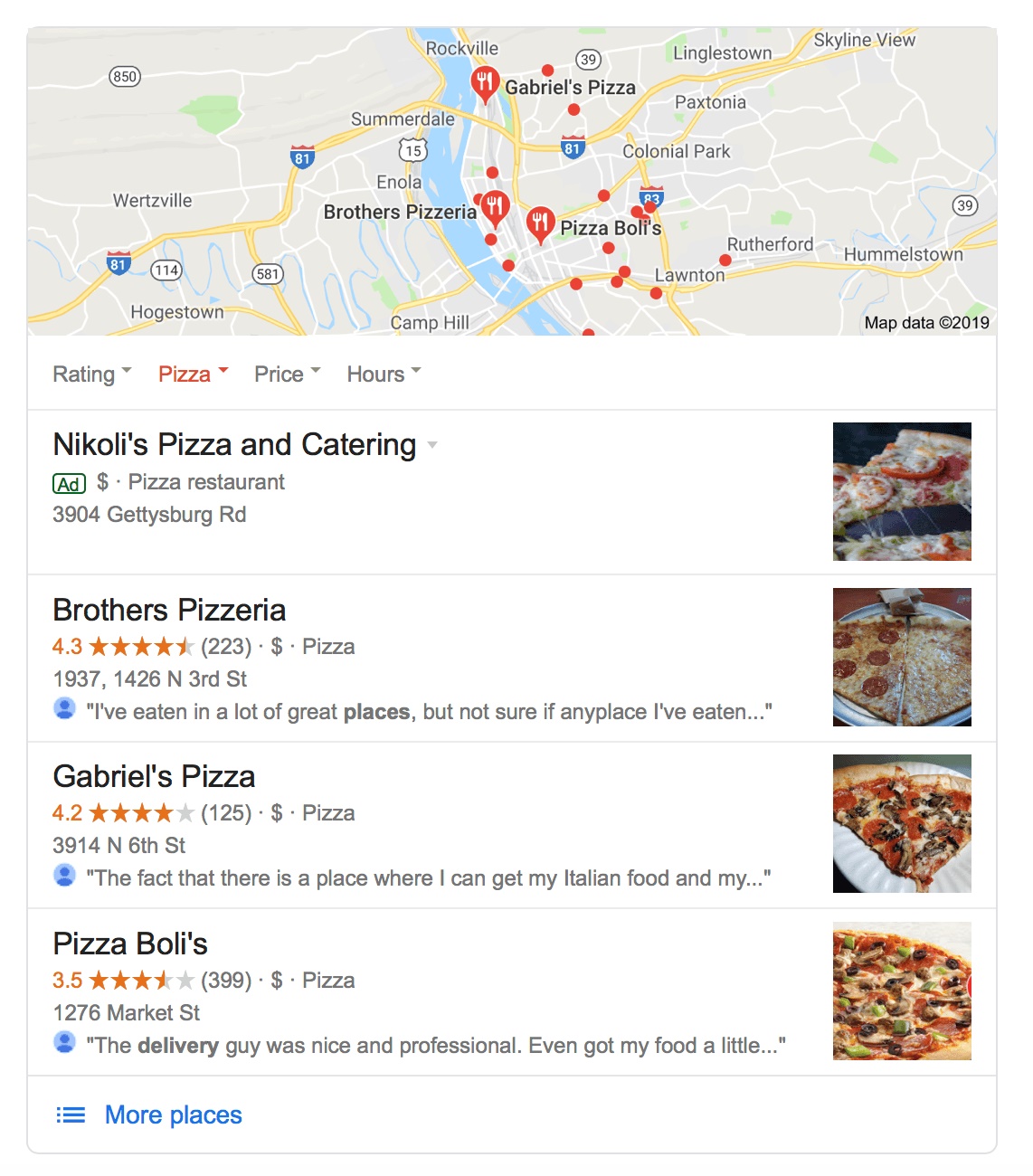At the top of the image, there is a map featuring various locations marked with map pins. The first marker at the top, indicated by a red pin, reads "Gabriel's Pizza" in bold black lettering. Another red pin in the middle marks "Brother's Pizzeria," and the last red pin towards the bottom points to "Pizza Boley's."

Below the map, the image has a white background with a header containing four tab options: "Rating," "Pizza," "Price," and "Hours." Each option has an arrowhead pointing downwards on the top right, signifying that they are clickable for more options. The "Pizza" tab is highlighted in red, distinguishing it from the others, which remain gray.

A thin gray line serves as a divider below the header. The first listing appears in bold black lettering and reads "Nicole's Pizza and Catering." To the right of this listing, there's an image of a pizza slice with stringy, white cheese stretching visibly. To the left, there's a small rectangular area outlined in green with the word "Add" in green text inside it. A single gray money sign (indicating price range) is shown in a bullet point, with "Pizza Restaurant" in small gray font beneath it. Below this text, it also says "3904 Gettysburg Road" in small gray font.

Another gray dividing line appears next, followed by "Brother's Pizzeria" in bold black text. To the right, there's an image of two slices of pizza—one slice is topped with pepperoni and the other with cheese, both plated on what appears to be either a paper plate or a white plate with a blue rim. To the left of this image, the rating is displayed as "4.3 stars" accompanied by an array of five stars, where around four and a half are filled in orange and the rest are gray. The number "223" is shown in small gray parenthetical text, indicating the number of reviews.